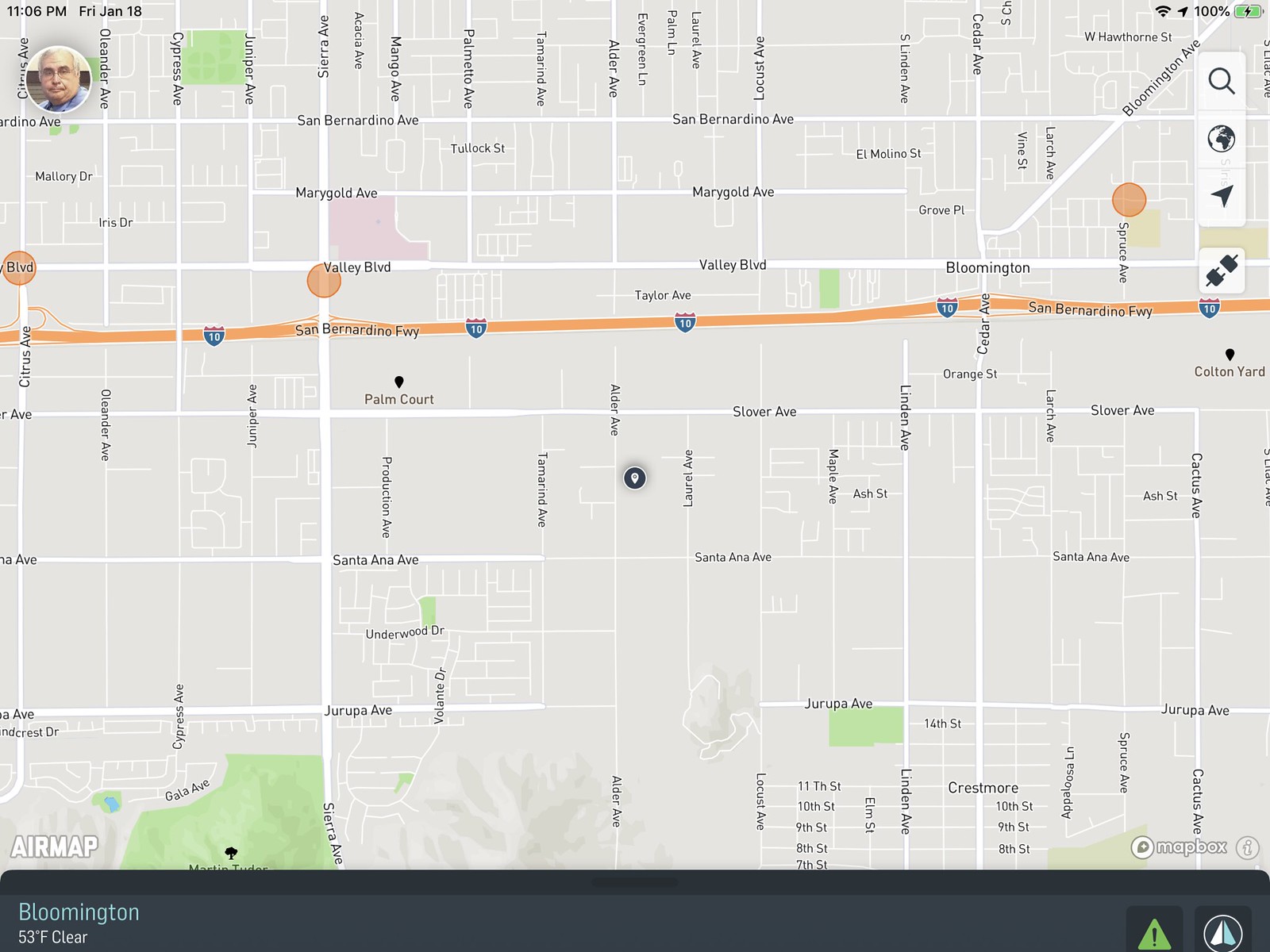The image features a detailed map centered on Bloomington, displaying a clear weather condition with a temperature of 53 degrees Fahrenheit in the bottom left corner. Below the weather information, there's a label that reads "Air Map." The top left corner of the map shows the date and time: Friday, January 18th, 11:06 p.m. Just beneath this, a small circular portrait of a man's face is visible. The map's primary focus is on Valley Boulevard and the surrounding streets that run parallel and adjacent to Interstate 10, which is clearly labeled. The intricate grid pattern of these streets is prominently displayed, highlighting their proximity to the San Bernardino Freeway.